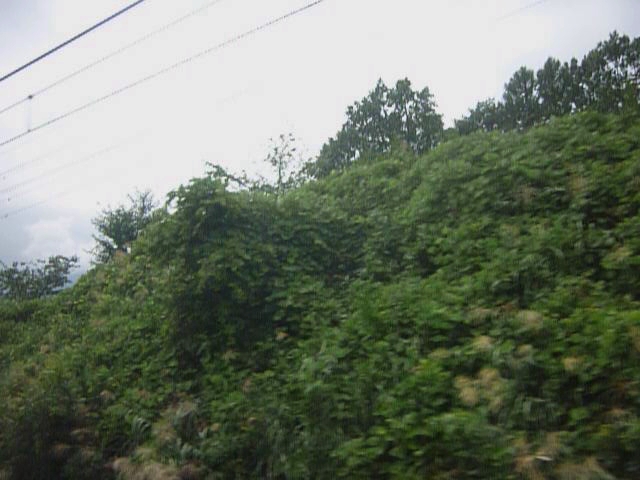The photograph depicts a blurred image, likely taken from a moving vehicle, of a lush tree line bordering a roadway or a steep bushy hillside. The upper left corner features several black overhead power lines, with three prominent lines clearly visible. The sky, which dominates the photo's upper part, transitions from a cloudy, evenly lit gray on the left to a possible diagonal blue hue reaching the middle. The foliage is dense and varied in shades of green, with hints of yellows and browns, adding to the impression of a vibrant but wild landscape. The foreground contains dry, grassy patches, and overall, the image exudes a desaturated, low-saturation aesthetic, suggesting an overcast or cloudy day.